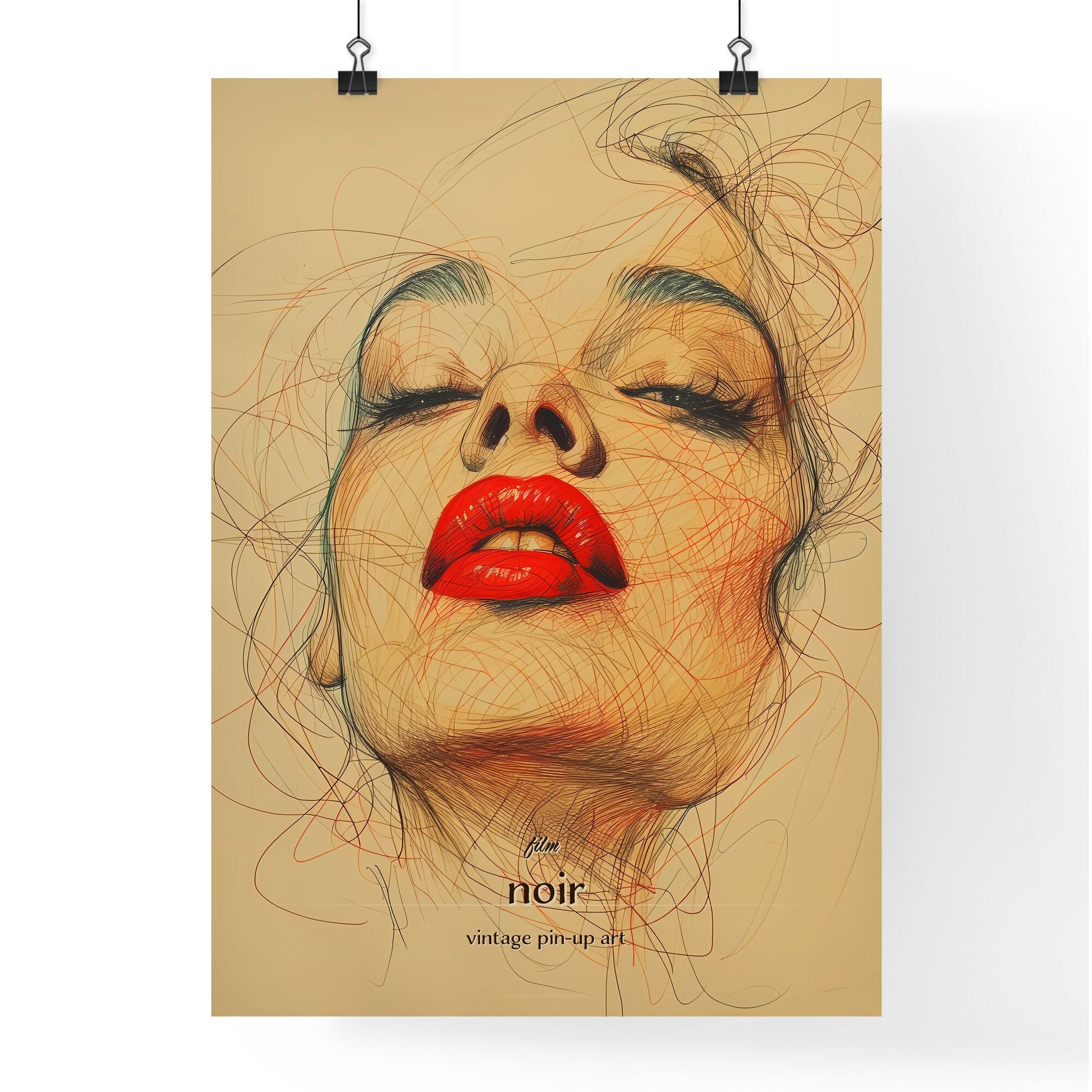The image primarily features a large poster or sign showcasing a striking artistic rendering of a woman's face. The detailed illustration, likely computer-generated due to its refined lines, suggests a blend of traditional and digital sketch techniques. The woman's chin and lips, vividly highlighted with bright red lipstick, command attention. Her two front teeth are visible, her nose is depicted from a lower angle revealing her nostrils, and her eyes are scrunched closed beneath long, prominent eyelashes. Dark black brows and possible eyeliner accentuate her expression, which seamlessly fades into a sepia-toned background at the forehead. Swirling lines, possibly representing her hair, add a dynamic element to the artwork. The poster is suspended by two clips and rope, and at the bottom, in clear text, it reads, "Film Noir Vintage Pinup Art." The color palette includes black, white, light brown, red, pink, and orange. This vivid, nostalgic piece appears suitable for display on a wall in a setting appreciative of vintage and artistic works.